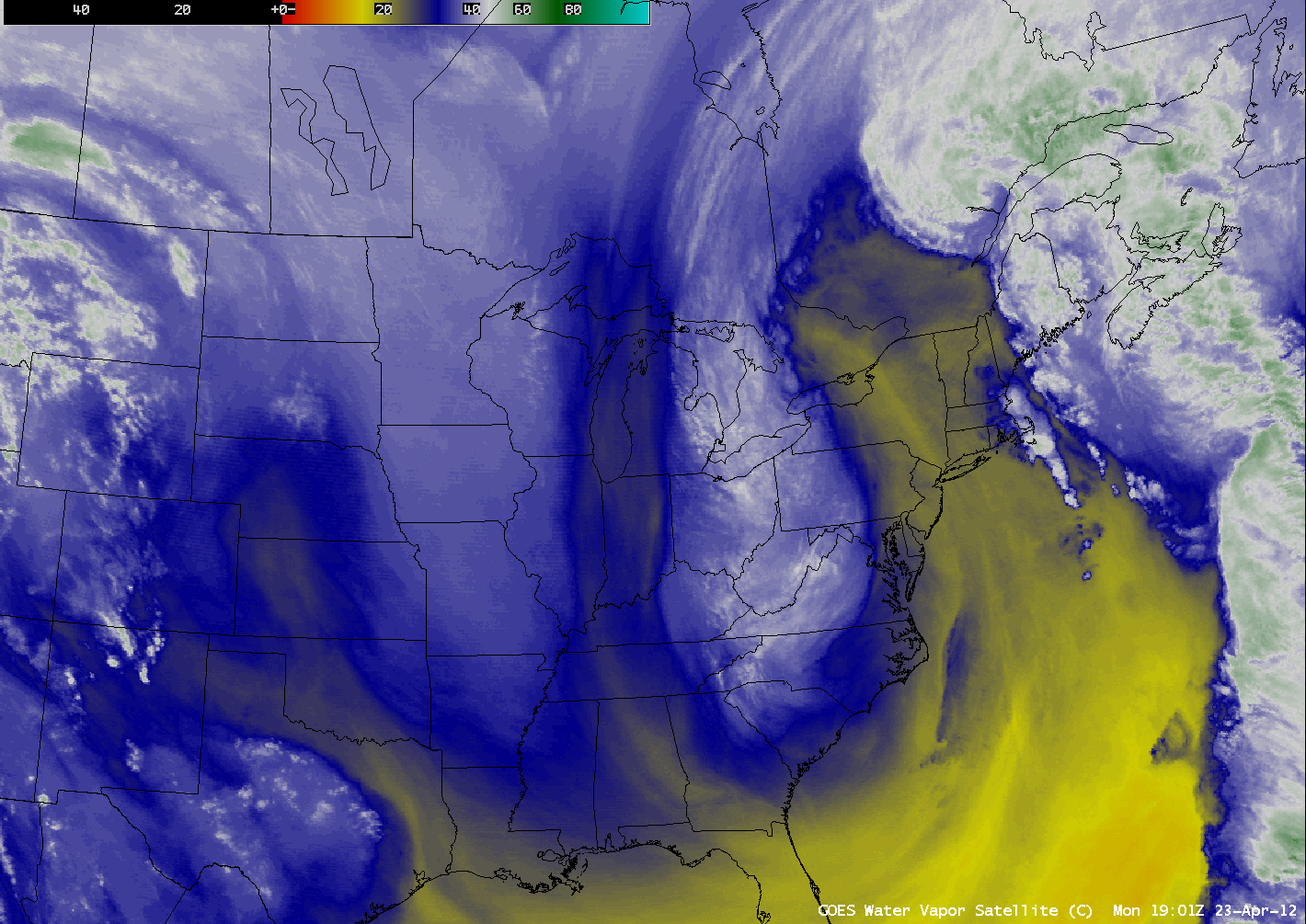This satellite image depicts water vapor patterns over the United States. The map is overlaid with black borders showing state boundaries and a color-coded bar in the top left corner that indicates water vapor intensity. The scale ranges from blue to yellow, with yellow indicating a high intensity. A prominent jet stream, colored bright blue, is also visible. A bright yellow water vapor cloud extends from Texas to New England, while toward Canada, the vapor turns white. Specific states like Kentucky, Ohio, Indiana, West Virginia, Virginia, Pennsylvania, North Carolina, South Carolina, Alabama, Georgia, Florida, Mississippi, and Louisiana are clearly visible. Cloud formations appear to swirl off to the west, with noticeable weather activity over Florida, Louisiana, Texas, and Oklahoma. Additionally, there are green and white cloud formations over the northeastern states and adjacent ocean areas. In the bottom right corner, the caption reads, "CCS Water Vapor Satellite," along with the date "Monday, 19, 012, 23, APR-12."